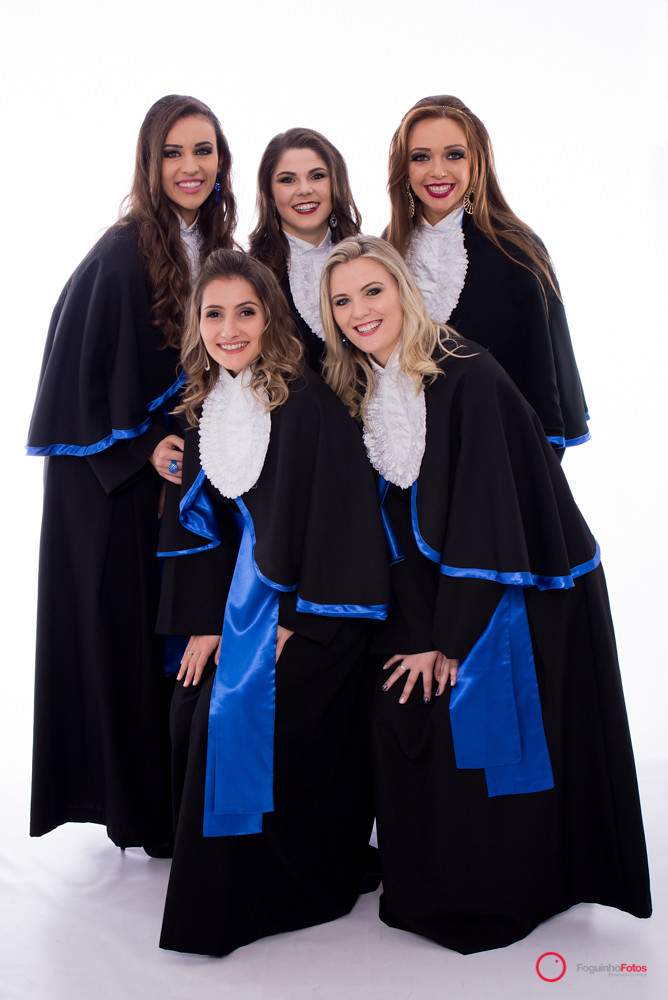In this vibrant portrait, five young women, likely in their late teens or early twenties, pose closely together against a white background, all smiling and wearing makeup including eye makeup and lipstick. The photograph captures a celebratory mood with the group dressed in identical black gowns that are adorned with a royal blue sash or ribbon, and featuring a decorative white piece around the neck, possibly suggesting legal symbolism. Each woman has long hair, reaching below their shoulders, with varying shades of brown and blonde. The three women at the back stand upright, showcasing different heights and hairstyles: the back-left woman has brunette hair, the middle has dishwater blonde or light brown hair, and the back-right woman has a more golden, blonde hue. In front, two women hunch slightly, their hands resting on their knees. The front-left woman has brunette hair, while the bottom-right has blonde hair and wears a distinctive blue ring on her finger. A red circle with the words "Bigger than photos" is visible in the bottom right corner, suggesting a possible affiliation with a singing group.